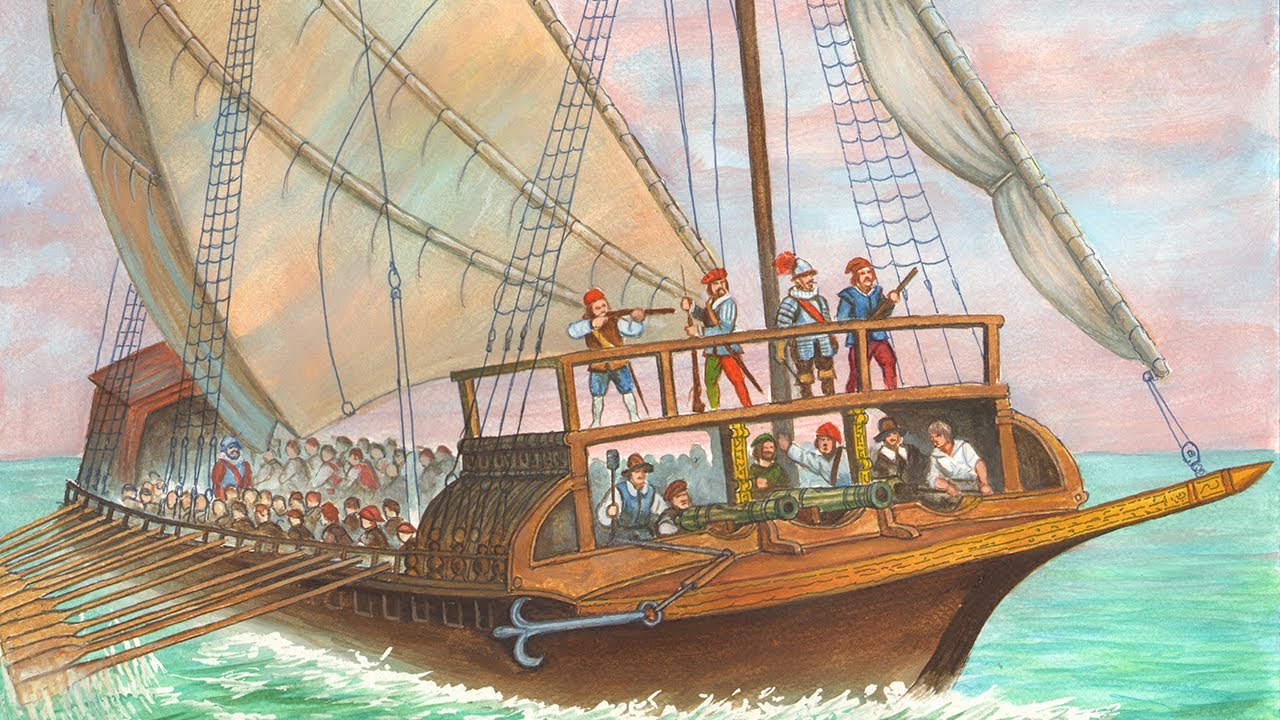This image is a detailed, hand-drawn illustration likely created for a book or textbook cover, titled "Naval Warfare in the Age of Sail" in a prominent yellowish-orange capital font against a gray overlay. The scene depicts an ancient wooden rowing ship from the 1700s or 1800s, rendered in a cartoon style. The ship is sailing on a teal-green ocean with frothy waves, beneath a picturesque sky painted in hues of pink and blue, suggesting dawn or dusk.

The vessel is constructed from light brown wood, with rows of long oars—at least ten on each side—extending from the sides. The ship’s structure features an open central section crowded with numerous men. At the prow, an anchor is visible, although not deployed.

At the front of the ship, two green cannons are mounted, manned by soldiers dressed in a mix of pilgrim-style and late 1700s to early 1800s uniforms, some wearing steel caps adorned with red feathers. On the upper deck, four men are seen: two wielding rifles, while one sports a silver hat with a red feather. The large mast on the ship supports white sails made of tan fabric, which are billowing in the wind, along with intricate netting.

Overall, the illustration captures the essence of an old-time sailing vessel powered by both sail and human effort, with a sense of readiness for naval combat.